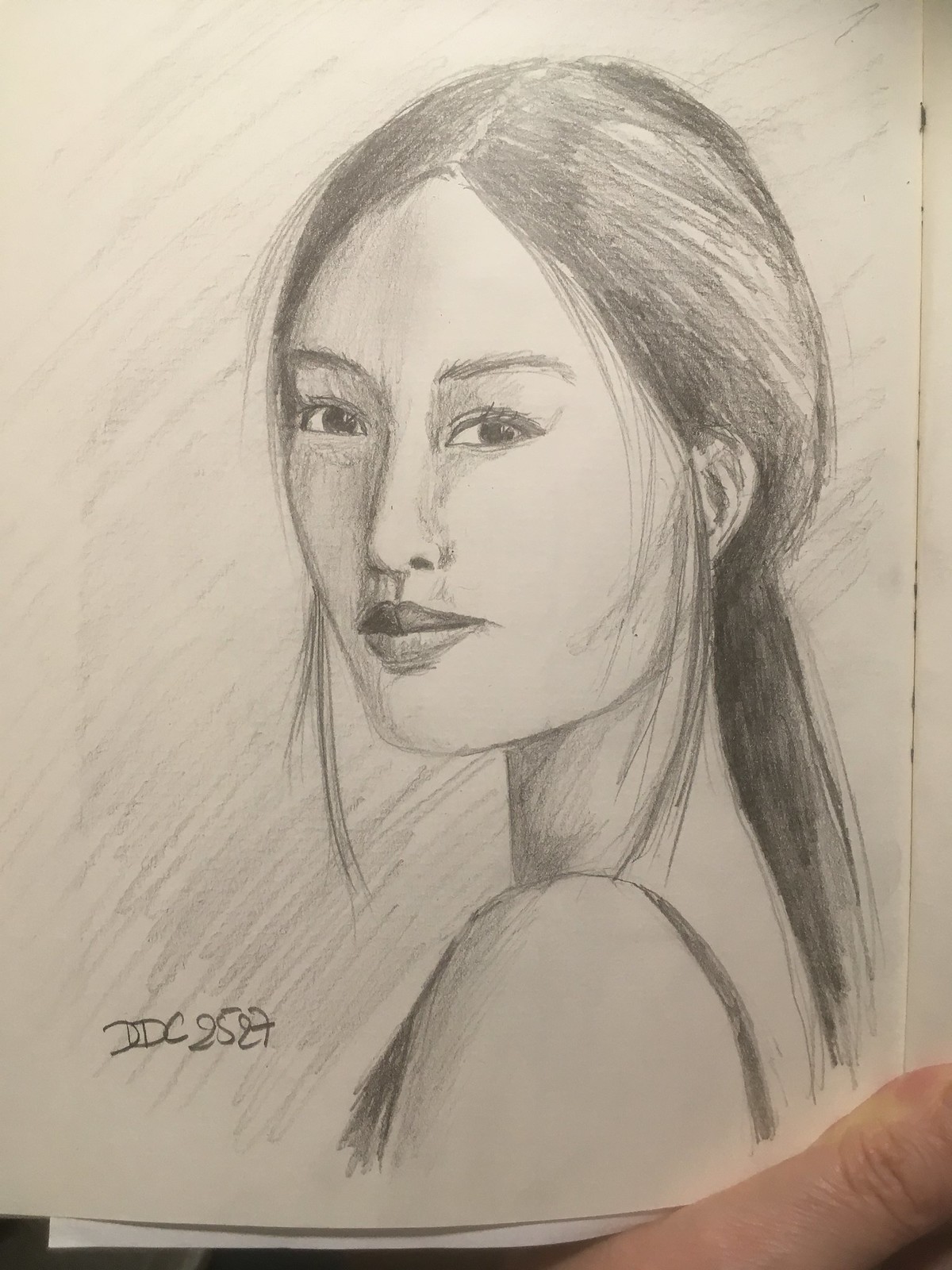A detailed pencil drawing on a rectangular sheet of paper, displayed in portrait orientation, captures a woman glancing back over her shoulder. Her hair is tied back in a low ponytail, and she wears a simple tank top, emphasizing the casual, yet intimate moment. The artistry is subtle and precise, with the artist’s initials delicately inscribed in the left-hand corner, adding a personal touch. The image of the drawing is being held by a hand, with part of the thumb visible in the bottom right corner, providing a sense of scale and human connection to the artwork.